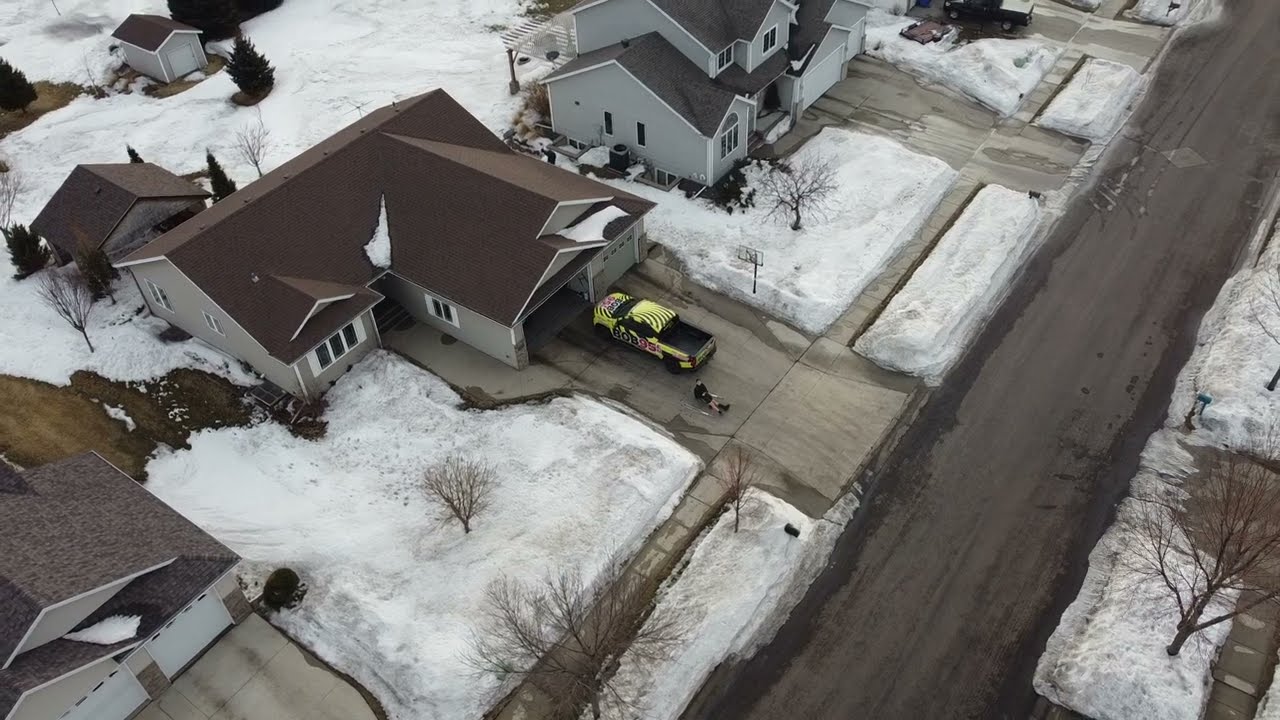The overhead drone image captures a snow-covered neighborhood subdivision with three distinct houses in the main focus. In the bottom left corner, there is a house with a gray roof. Diagonally above it towards the center, there's a house with a reddish-brown roof, complete with a driveway where a yellow pickup truck with graphics, possibly a work truck, is parked in front of an open garage. To the right of this house is another home with a gray roof, a snow-covered yard, and a tree in the front. The streets, sidewalks, and driveways have been cleared of snow, and the overall scene is set against an overcast sky, suggesting it might be early morning or evening. The image also hints at the presence of additional houses and sheds in the background.